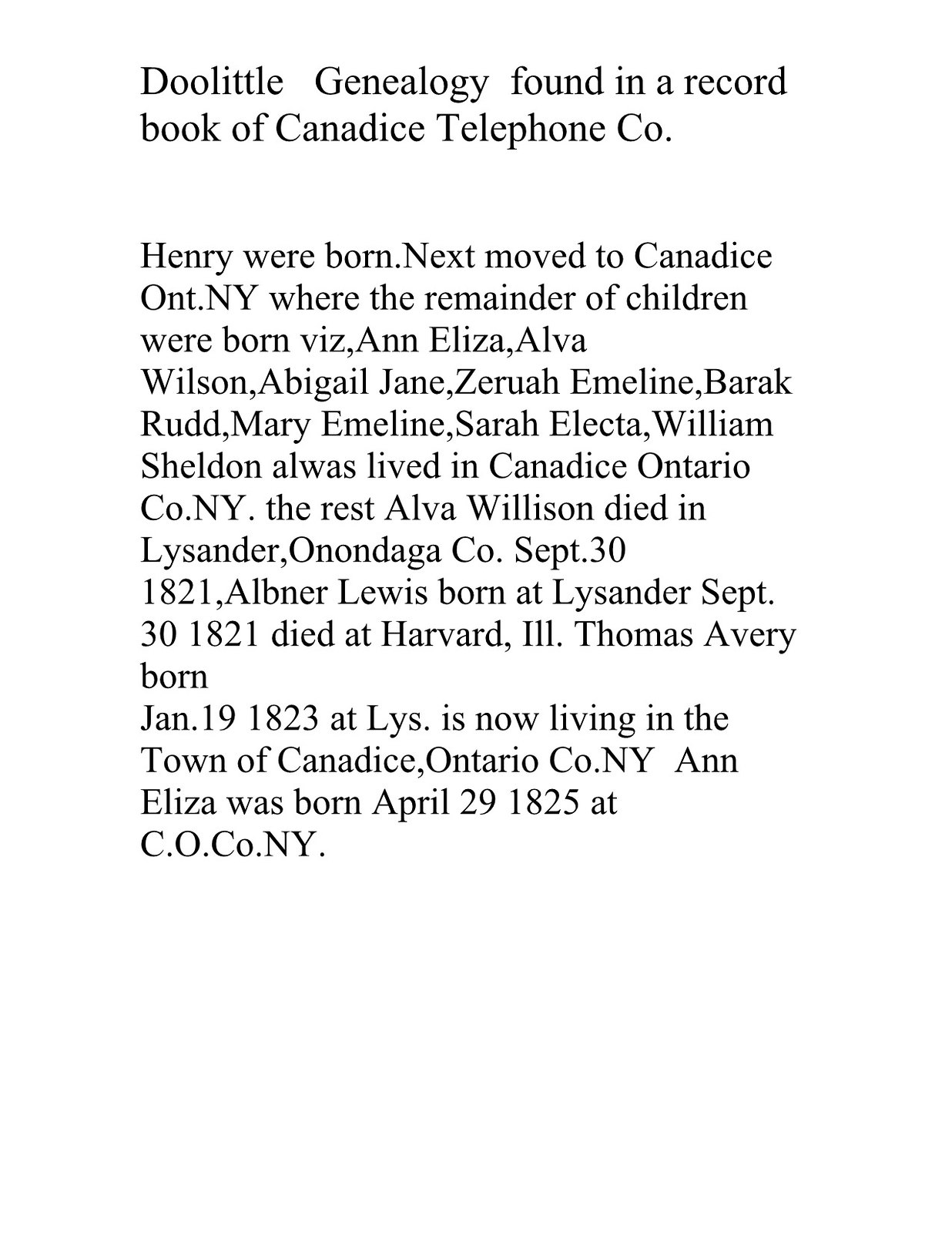The black Times New Roman text on a white background begins with "Doolittle Genealogy," a title found in a record book from the Canadice (spelled C-A-N-A-D-I-C-E) Telephone Company. It details the lineage of the Doolittle family, starting with Henry, who was born and subsequently moved to Canadice, Ontario County, NY, where the remainder of the children were born. The children listed are Anna Eliza, Alva Wilson, Abigail Jane, Zeruah Emmeline, Barak Rudd, Mary Emmeline, Sarah Electa, and William Sheldon, all of whom reportedly lived in Canadice, Ontario County, NY. Alva Wilson died on September 30, 1821, in Lysander, Onondaga County. Abner Lewis, born in Lysander on the same date, later died in Harvard, Illinois. Thomas Avery, born January 19, 1823, in Lysander, is now residing in Canadice, Ontario County, NY. Anna Eliza was born on April 29, 1825, also in Canadice, Ontario County, NY.